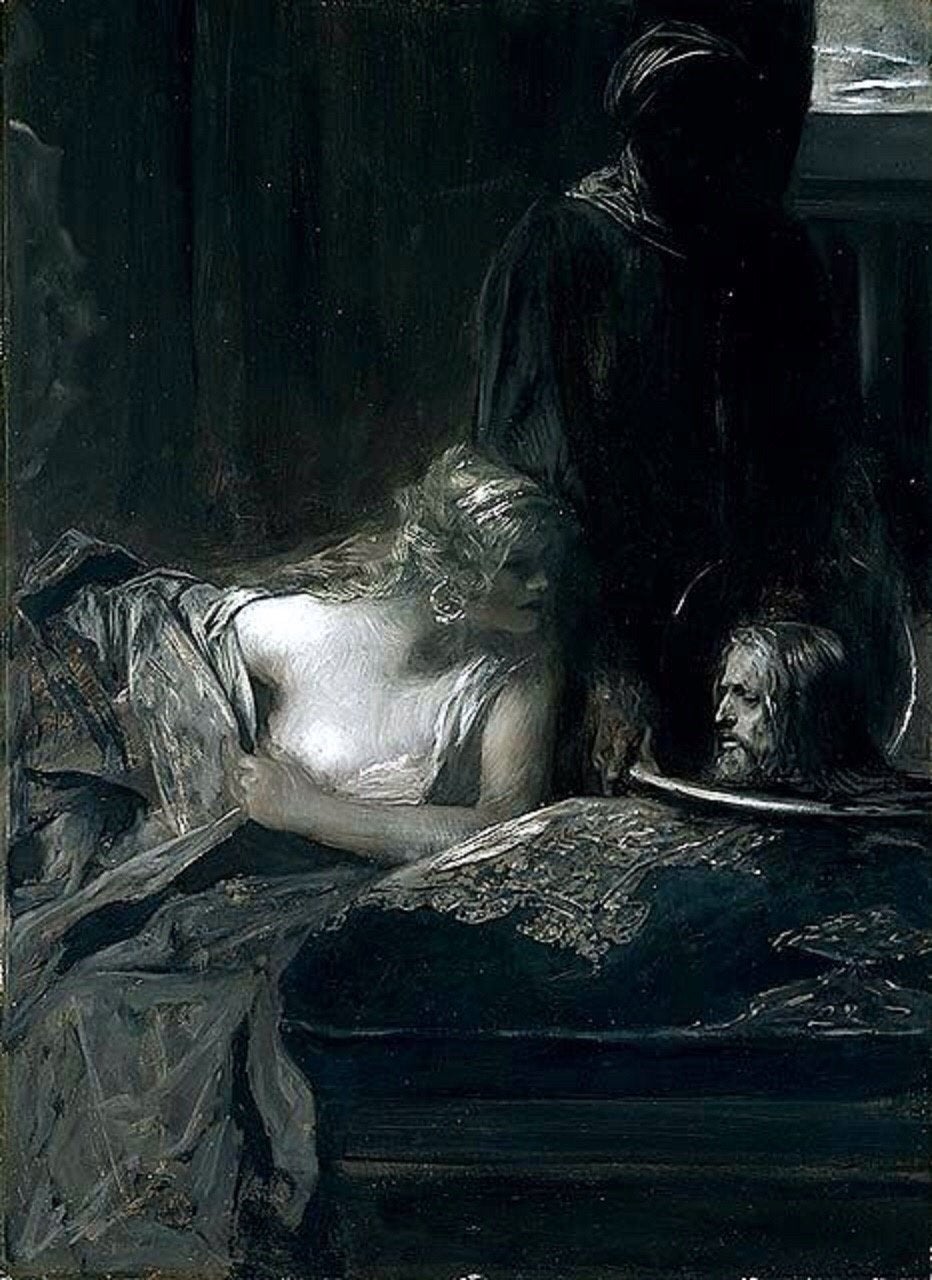The image is an oil painting that showcases a dramatic and somewhat eerie scene, blending realistic and stylistic elements. Central to the composition is a woman with curly blonde hair and very light skin, draped in white and gray robes. She leans over a large, black cushion adorned with ornate silver-brown designs, her gaze directed to the right. Resting on this cushion is a circular metal tray that holds the disembodied head of a man. The man's head has light skin, a pronounced nose, long black hair, and a beard, giving him a solemn or perhaps serene expression, as if he is sleeping.

Standing behind the cushion and tray is a tall, cloaked figure dressed entirely in black. This figure's face and head are completely obscured, shrouded in shadow, adding a mysterious and foreboding presence to the scene. The setting appears to be indoors, enveloped in a dark and textured background with subtle vertical lines, possibly indicating curtains or a patterned wall. The overall coloration of the painting is dominated by muted tones, contributing to the somber and gothic atmosphere, with the focus drawn starkly to the contrasting lightness of the woman's attire and the man's head.